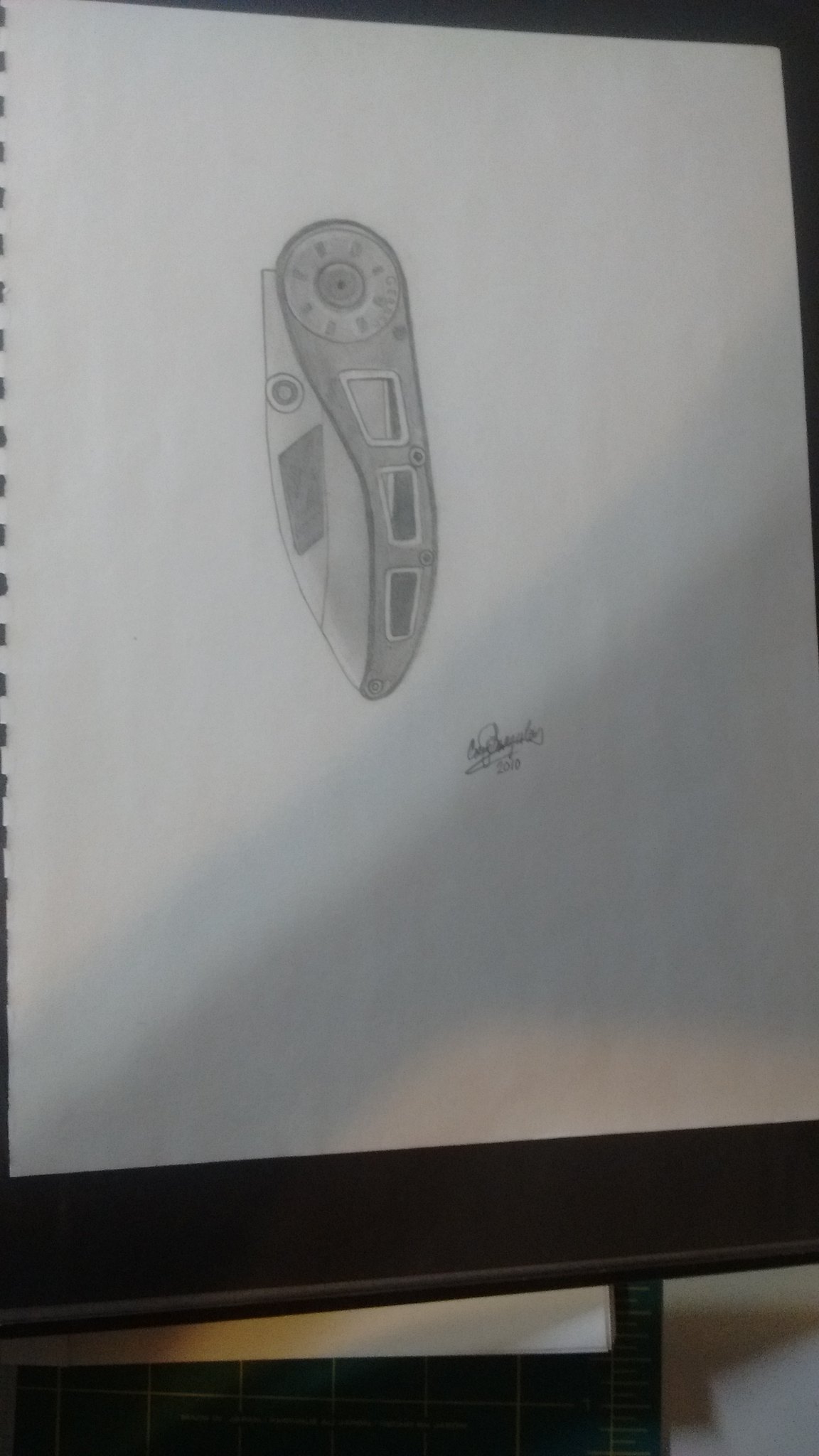The image depicts a detailed pencil sketch on a large piece of white spiral-bound sketch paper, propped against a dark wooden drawing board. The central figure in the drawing resembles a folded switchblade knife, characterized by a curved casing and intricate shading. The blade, discernible on the left side, features a circular element coupled with a parallelogram shape, while the handle displays four smaller rectangular shapes. Below the sketch, the artist's signature is visible, along with the year "2010." At the photo's bottom, a green ruler with white lines lies beneath a thick, solid brown bar, adding depth to the composition.